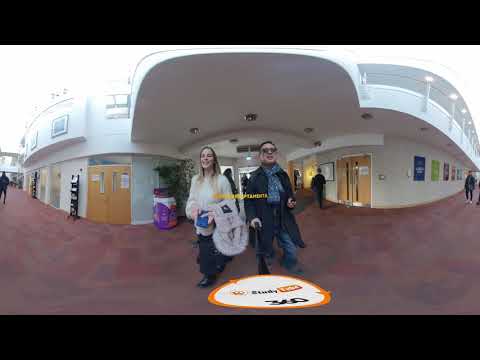In the photo, two individuals stand prominently in front of a unique white building characterized by its distinctive beveled roof and large awning adorned with lights. The building has prominent brown doors. The left side of the image features a blonde woman with long, chest-length hair. She is wearing a white, long-sleeved sweater under a furry jacket draped over her left arm, paired with dark pants and dark shoes. She holds a blue container and is smiling. To her right is a man with short dark hair and a darker complexion, suggesting he may be of Asian descent. He wears dark sunglasses, a long black trench coat, a blue scarf, and jeans. In the foreground, there's a distinctive white circle with orange trim on the ground, containing the number 360 and the word “study.” To the left side of the scene, there is a purple trash can, and both sides of the photo show hallways with people walking along them, hinting at a lively atmosphere, possibly near an elevator or within a hotel.